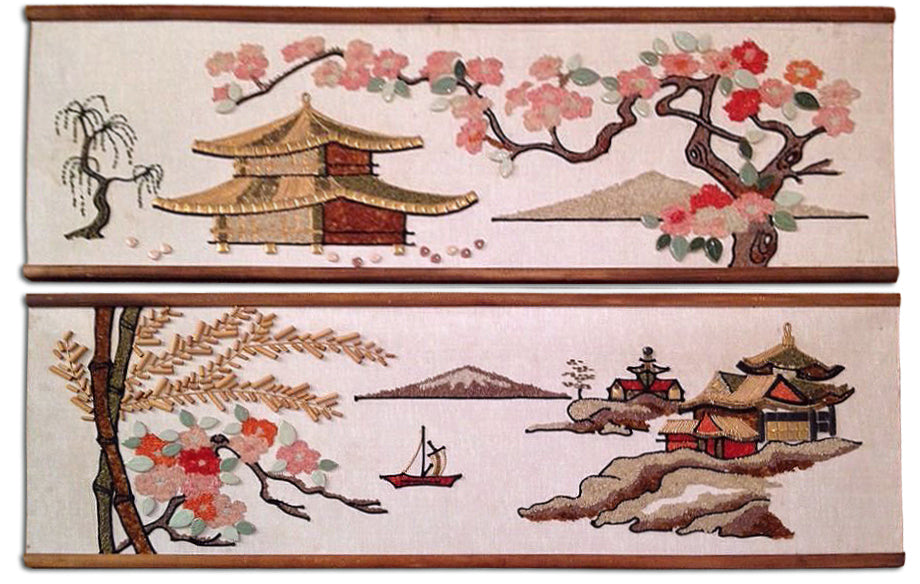The image showcases two horizontally laid out Japanese-style art pieces, each mounted on wooden rods at both the top and bottom. The artworks, which appear to be either painted or embroidered on grey or beige fabric, feature intricate depictions of traditional Japanese scenes. 

In the top painting, on the left side, a tree with shady, drooping leaves is visible next to a pagoda-like building with two decks, rendered in shades of brown. Across from the building, on the right side, a tree branch is adorned with a medley of pink, red, and white cherry blossoms, set against the backdrop of a small hill in the distance.

The bottom artwork showcases a more expansive landscape. On the left side, tall branches with vibrant yellow leaves and red-pink flowers stretch into the sky. On the right side, several buildings with pagoda-like architecture are positioned next to a small hill, reinforcing the scene’s Japanese setting. Additionally, a boat situated in the middle of the composition highlights the cultural motif, aligning with Japan's rich maritime traditions and seafood industry. Overall, the art pieces evoke a serene and picturesque representation of traditional Japanese landscapes, complete with cherry blossoms and iconic buildings.